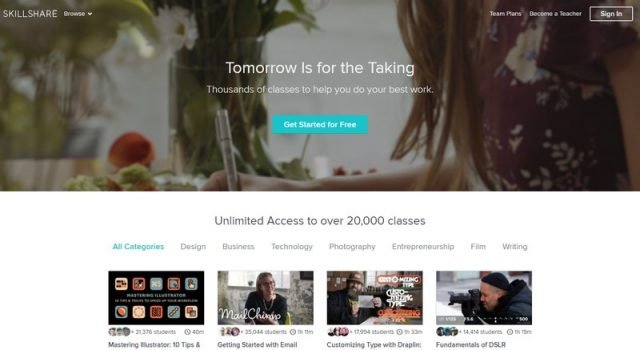This photograph captures the homepage of the Skillshare website. In the top left corner, a light gray "Skillshare" logo is prominently displayed, followed by a "Browse" option with a dropdown arrow, likely for navigation. The background of this header section depicts a woman with long hair, whose face is not visible. She wears a maroon red floral shirt adorned with yellow, white, and pink flowers cascading down the front and side. She holds a white pen in her hand and has light skin. 

In the scene, there is a vase of white flowers with yellow centers and deep green leaves positioned both to her right and in front of her. Some flowers are also visible on the table, though partially cut off by the photograph’s edge. 

On the far right of the header section, text reads "Team Plans" and "Become a Teacher," next to a semi-transparent button bordered and texted in white that says "Sign In." 

Centrally, the bold white text proclaims, "Tomorrow is for the Taking," followed by a subheading, "Thousands of Classes to Help You Do Your Best Work." Below this, a teal button with bold white text invites users to "Get Started for Free."

Outside this main banner, bold black text announces, "Unlimited access to over 20,000 classes," followed by a list of selectable categories. The first category, highlighted in teal blue, reads "All Categories," followed by "Design," "Business," "Technology," "Photography," "Internship," "Film," and "Writing," each in standard black text.

Below these categories, various images represent different classes. One image, partially cut off, reads "Mastering Illustrator: 10 Tips." Another shows a woman in a living room with the text "Getting Started with Email." A third image features a man with a thick beard and brown hat, holding a piece of paper, under the title "Customizing Type with Droplet." The last image depicts a man in a heavy coat and toboggan, holding a black camera, under the caption "Fundamentals of DSLR."